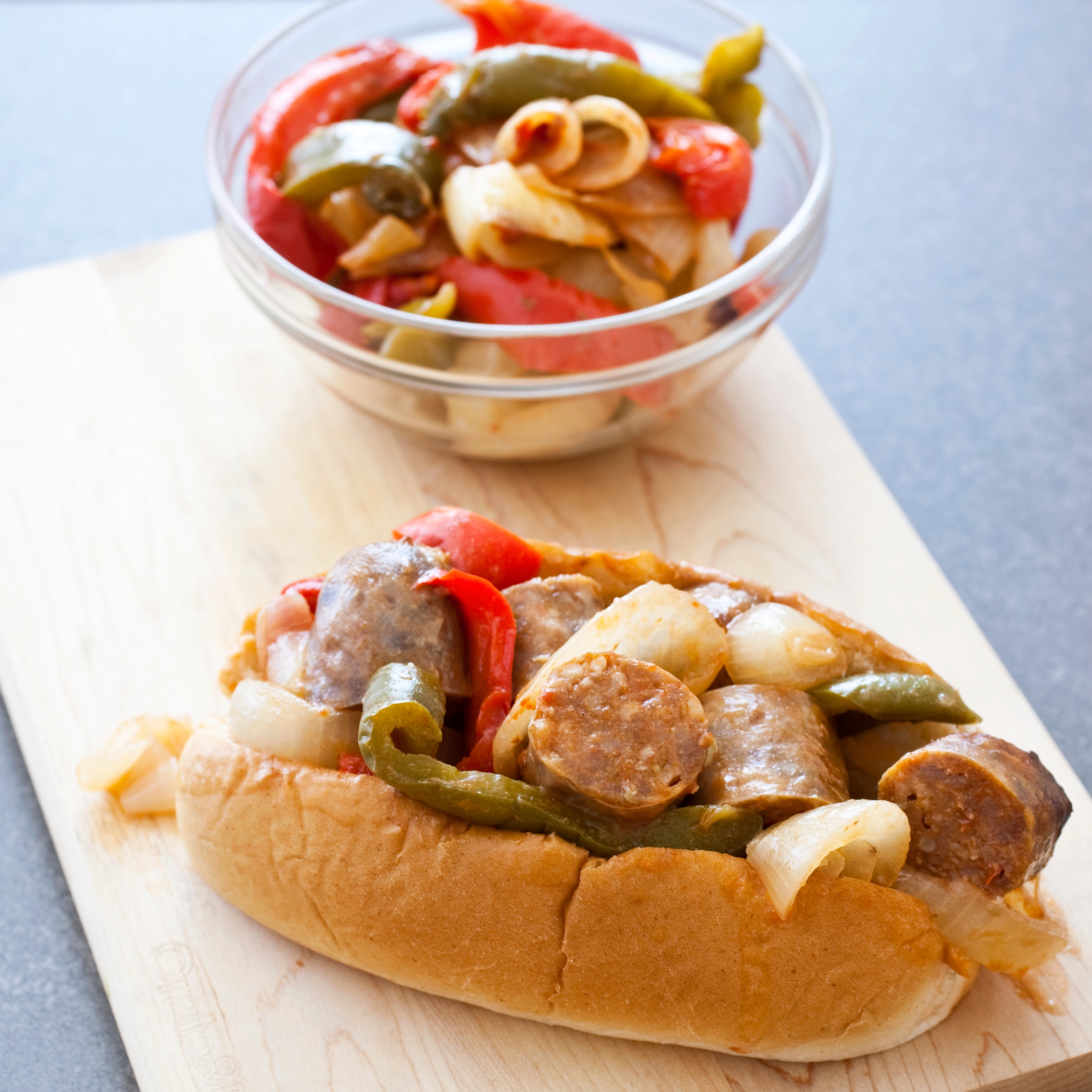The image depicts a meal centered around a sandwich that features a sausage, possibly overcooked, nestled within a fresh hoagie bun. The sausage is complemented by grilled or sautéed red and green bell peppers and onions. This sandwich is presented on a light brown wooden cutting board situated on a gray table. In the background, there is a small clear bowl containing a mix of the same grilled peppers and onions, hinting at additional toppings or ingredients. The overall appearance suggests a home-cooked meal, albeit with a slightly unappetizing-looking sausage.